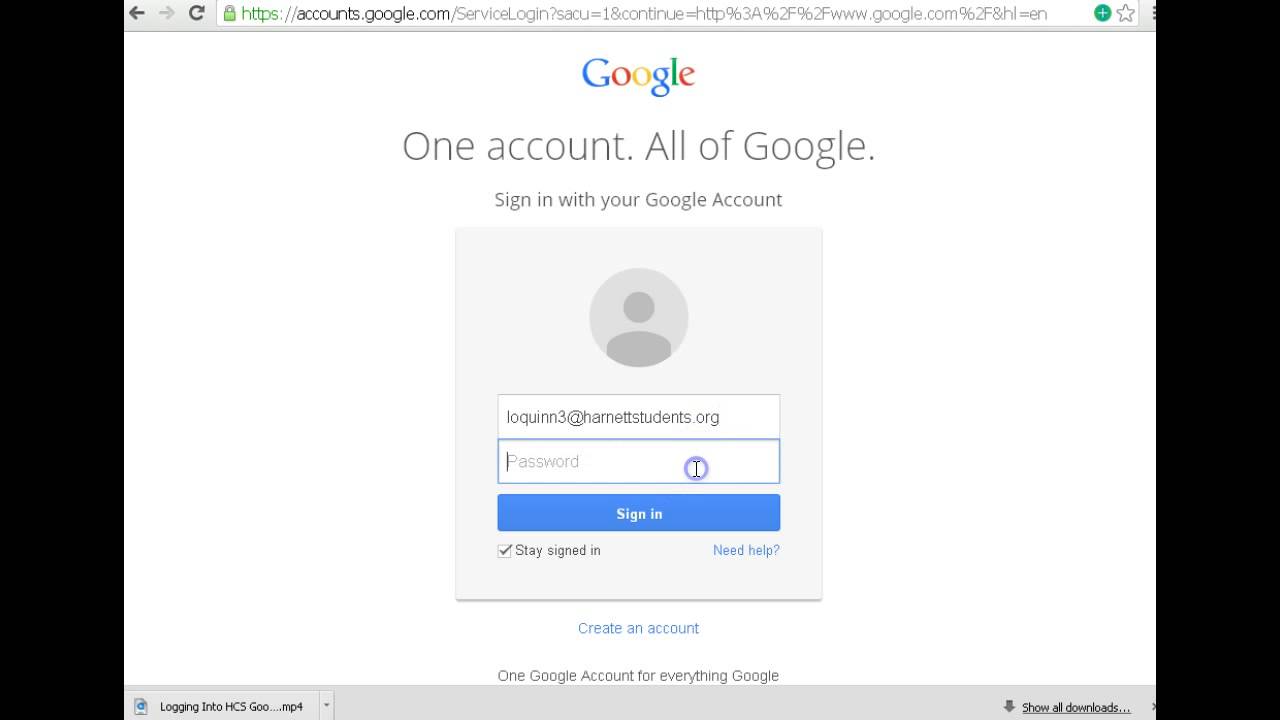This image is a screenshot displaying the Google account login page within a web browser. At the top center of the image, the address bar shows that the user is currently on "account.google.com." In the top left corner, there are navigation buttons including a forward button, a back button, and a reload button. On the top right, there is a settings button for browser configurations and a gray star for adding the webpage to the favorites or bookmarks.

Dominating the center of the image, the main portion of the screenshot, is the Google account login page with a white background. Positioned at the top center of this section is the Google logo in its iconic red, blue, yellow, and green colors. Below the logo, grey text reads, "One account. All of Google." Reinforcing the purpose of the page, further text instructs, "Sign in with your Google account."

In the middle of the page is a light grey box, featuring a silhouette of a person to denote the user's profile picture. Below this silhouette is an input field pre-filled with the email address "loquin3@harnettstudents.org." Adjacent is another input field requesting the user's password. At the bottom of this grey box is a blue button with white text that says, "Sign in," which, when clicked with the correct credentials, will log the user into their Google account.

Beneath this sign-in section, there's a blue link labeled "Create account," offering users the option to create a new Google account. Further down, black text states, "One Google account for everything Google," hinting at the extensive services accessible through a single login. Additional detailed information about the Google account is available as the page extends below this initial login interface.